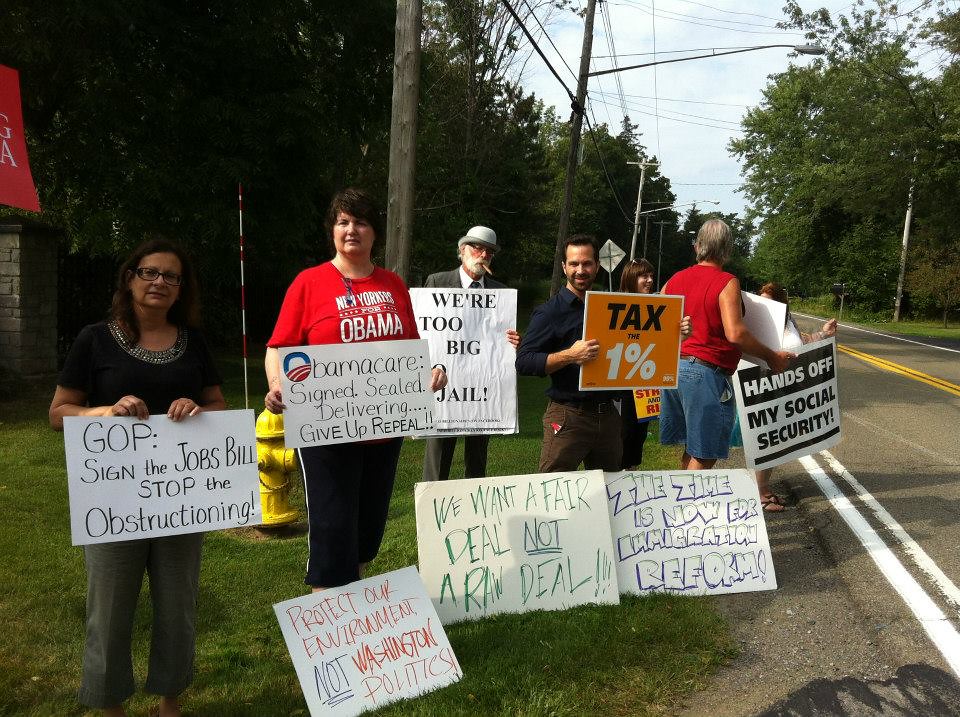The photograph depicts a diverse group of male and female protestors standing on the grassy shoulder of a two-lane road, marked by double yellow stripes in the middle and white edge lines, some of which are slightly encroached upon by their signs. The backdrop includes a treed area with light poles and telephone poles. The protestors hold an assortment of signs advocating for various issues. Prominent among them are signs that say, “GOP, sign the jobs bill, stop the obstruction,” “Obamacare: sign, seal, deliver, give up, repeal,” and “We want a fair deal, not a raw deal, we're too big for jail.” Additionally, one protestor is dressed as the Monopoly man, complete with a cigar, and another holds a sign demanding "Tax the 1%." Other visible signs include "Hands off my Social Security" and "The time is now for immigration reform." The diversity of the signs indicates a protest addressing multiple grievances and calls for action on several fronts.